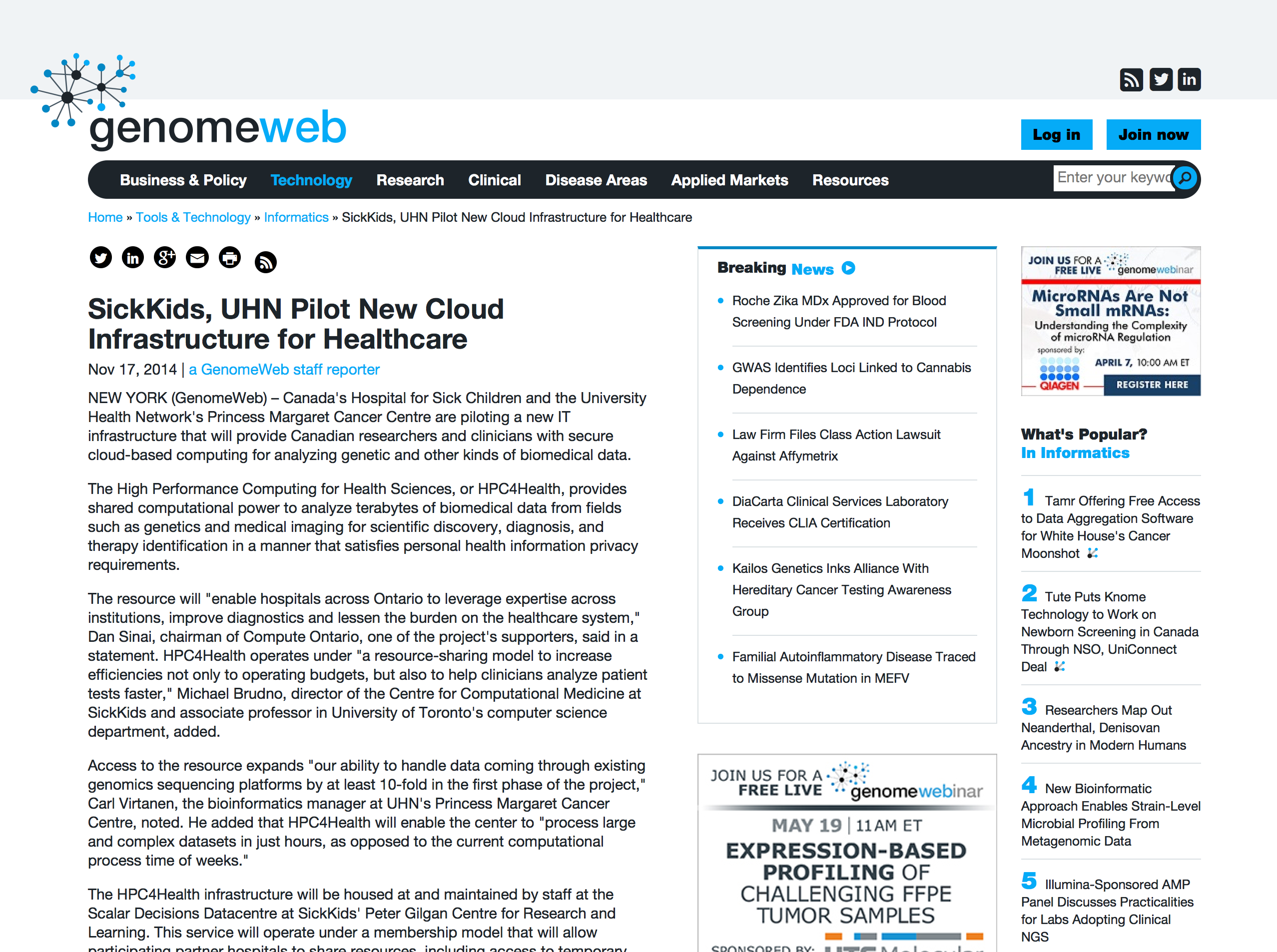**Website Interface Description**

In the top left corner of the web page, there is a gray horizontal bar displaying the Wi-Fi icon followed by the Twitter and LinkedIn icons. Beneath this gray bar, a white strip features the text "Genome Web" with "Genome" in black and "Web" in blue, accompanied by options to "Log in" or "Join now."

Below this, there is a black navigation bar that organizes the site’s main content into several categories, such as "Business and Policy" in white text, "Technology" in blue, and "Research," "Clinical," "Disease Areas," "Applied Markets," and "Resources" all in white letters. A white search bar sits beneath the navigation bar, distinguished by a black magnifying glass icon inside a blue circle.

The main content area features the page’s headline: "Home, Tools and Technology, Information, Sick Kids, UHN, Pilot New Cloud Infrastructure for Healthcare," dated November 17, 2014. On the right side of this section, a "Breaking News" headline invites users to join a free live Genome webinar titled "Expression-based Profiling of Challenging FFPE Tumor Samples."